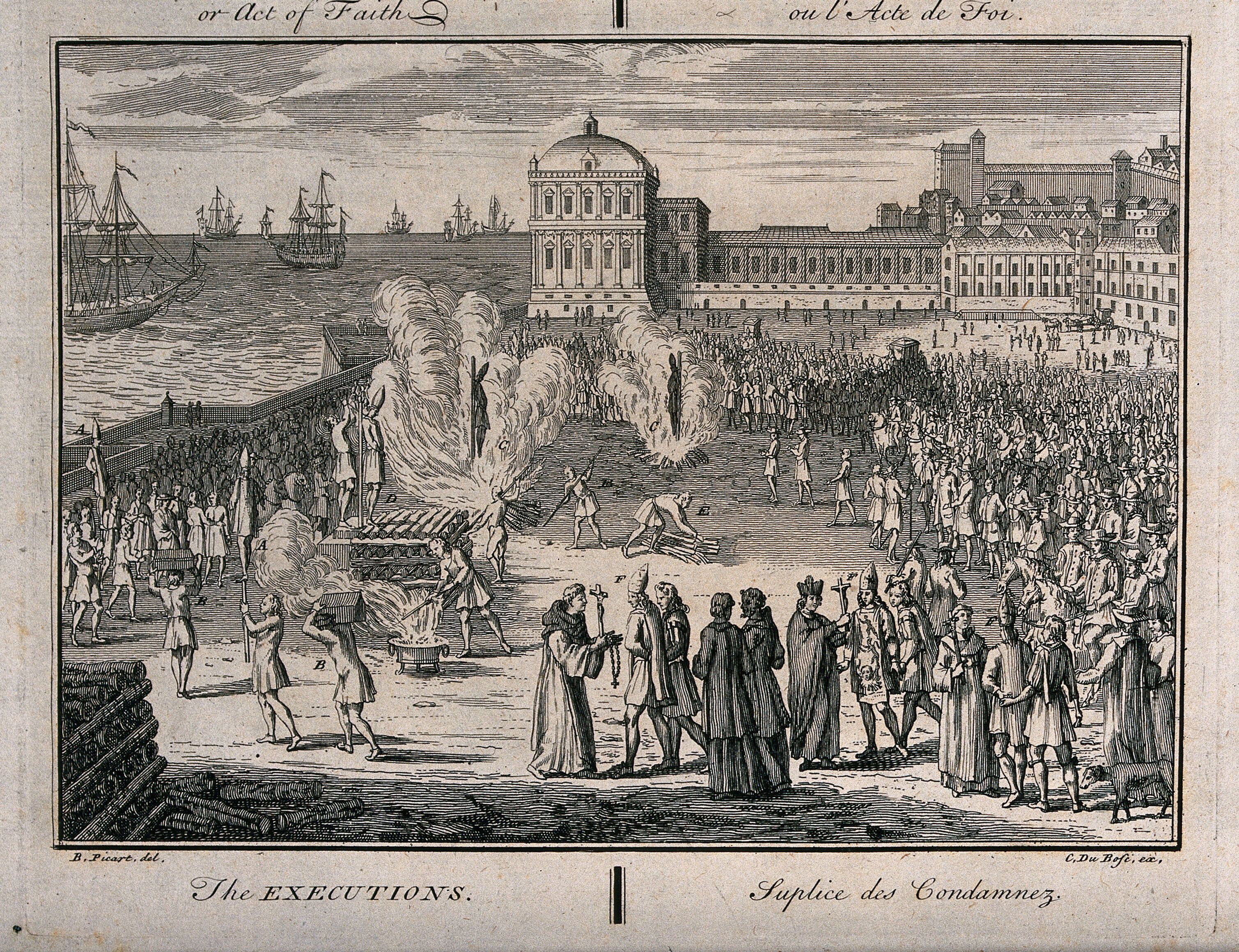This intricately detailed old black-and-white sketch, aged to a pinkish gray hue, features an image of solemn gravity. Measuring approximately six inches wide by four inches high, the rectangular piece is bordered in black with inscriptions at the corners. The top left reads "Act of Faith" in English, mirrored on the top right in French as "L'acte de foi." Similarly, the bottom left is labeled "The Executions," with its French counterpart "Suplice des Condamnes" on the bottom right.

The complex scene within depicts a fenced-off area teeming with people. On the right side, a dense crowd includes religious figures and servants carrying trays and buckets, while in the background, castle-like buildings or town structures loom. The sketch graphically portrays the dire reality of its title: people are shown handcuffed or shackled, and in the distance, some are being hung and burned alive, engulfed in fire and smoke. On the left side, there is a stark contrast with tranquil waterfront imagery featuring numerous sailboats, demarcated by a wall that separates the chaotic land scene from the calm sea. The profound juxtaposition within this historic drawing encapsulates a chilling narrative of faith and mortality.